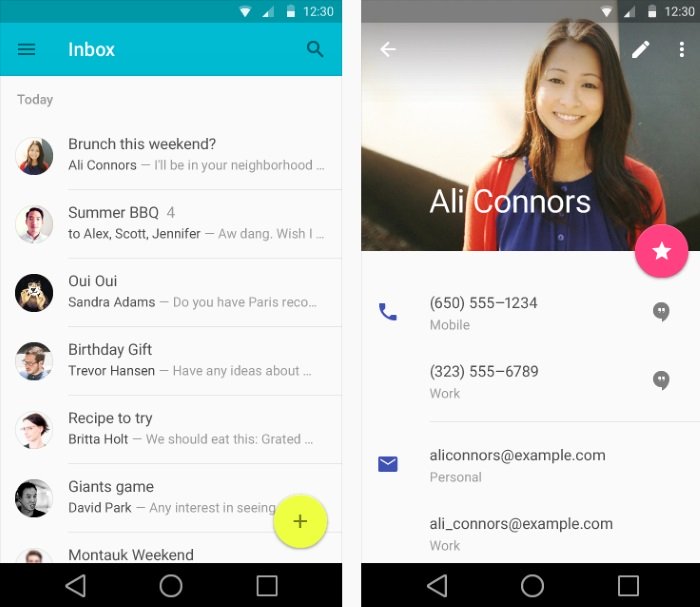**Detailed Caption for Image:**

The image consists of two smartphone screenshots placed side by side. The screenshot on the left displays an email inbox interface. At the top of this screenshot, there are standard status icons indicating Wi-Fi connectivity, signal strength, battery level, and a timestamp showing 12:30. Below this, a navigation bar features a hamburger menu on the left and a search icon on the right, with the word "Inbox" centered between them.

The inbox lists seven emails, each accompanied by a user photo. The first email is titled "Brunch this weekend" from Oli Connors, with the preview text "I'll be in your neighborhood." The second email, "Summer Barbecue 4," is addressed to Alex, Scott, and Jennifer. Following that is an email from Sandra Adams titled "OuiOui," with the preview text "Do you have Paris Rico..." The fourth email, "Birthday gift," is from Trevor Hansen and previews with "Have any ideas about..." Next is "Recipe to try" from Britta Holt, with the text "We should eat this, grated..." The sixth email is titled "Giants game" from David Park, with the preview "Any interest in seeing?" The final email, "Mind Talk Weekend," is partially cut off with a visible plus sign.

The screenshot on the right provides a detailed view of a contact, presumably after selecting Oli Connors from the inbox. This interface retains the same top status icons and navigation bar as the inbox view but includes a left-facing arrow for navigation back, a photograph of Oli Connors, a pencil icon for editing, and three vertical dots for additional options. Below Oli Connors's image, there is a star icon followed by his contact details, including a mobile phone number, work phone number, email addresses, and both personal and work addresses.

Both screenshots feature navigation buttons at the bottom, including left-facing arrows, home buttons, and stop buttons.

These comprehensive descriptions highlight the layout and specific details contained in each part of the interface depicted within the screenshots.